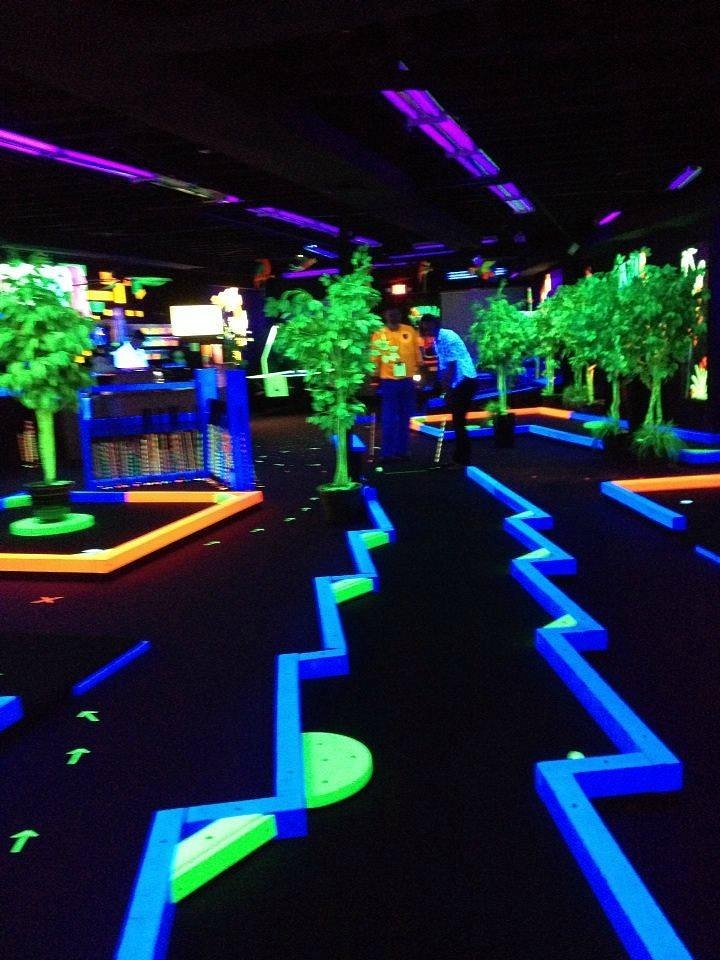The photograph captures a vibrant glow-in-the-dark mini-golf course illuminated under black lights, transforming the typical game into an electrifying experience. Central to the image are two people standing at the edge of one of the mini-golf holes, each holding a club. The individual on the right wears a blue shirt and black pants, while the person on the left dons an orange shirt paired with blue pants, both glowing brightly under the black light. The course is adorned with vividly green trees that stand out strikingly against the black backdrop. Additionally, the floor features blue zigzag paths, and the ceiling is decorated with strips of purple and pink lights, heightening the game's immersive atmosphere. Off to the sides, more sections of the course are visible, and in the background, a concession stand and some screens can also be seen, completing the lively setting.